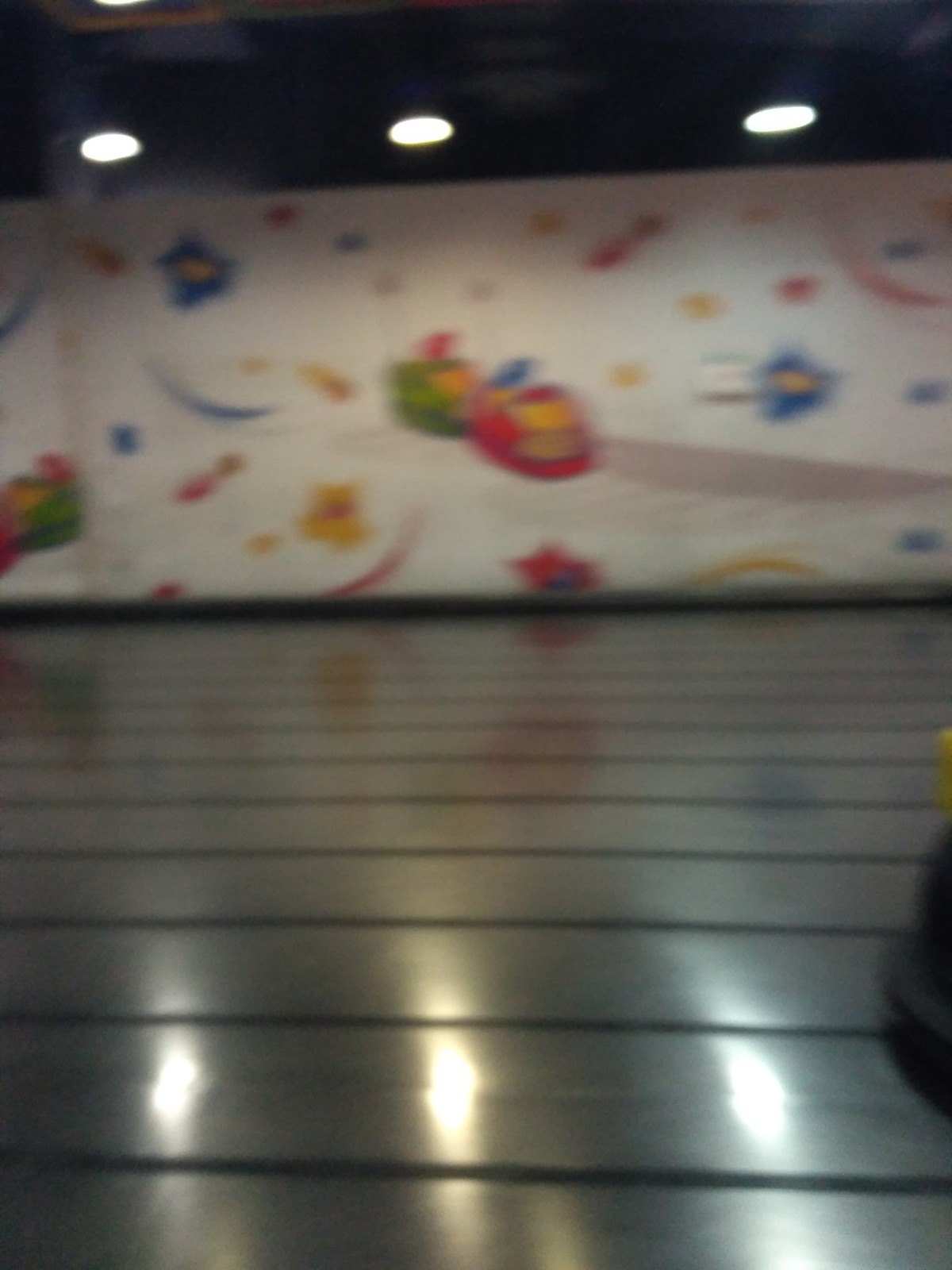A blurry photograph captures the dynamic energy of an indoor amusement park. Despite the motion blur suggesting high-speed action, various details are discernible. At the back, a large white banner, adorned with stars and cartoonish go-kart illustrations, sets the playful scene. The bottom right corner of the image hints at a go-kart, partially cut off, implying the presence of a go-kart track. The floor, reflecting the light, is a shiny black and grey, adding to the sleek, modern ambiance. Overhead lights on the ceiling illuminate the otherwise dark surroundings, enhancing the vibrant atmosphere typical of a children’s amusement park.